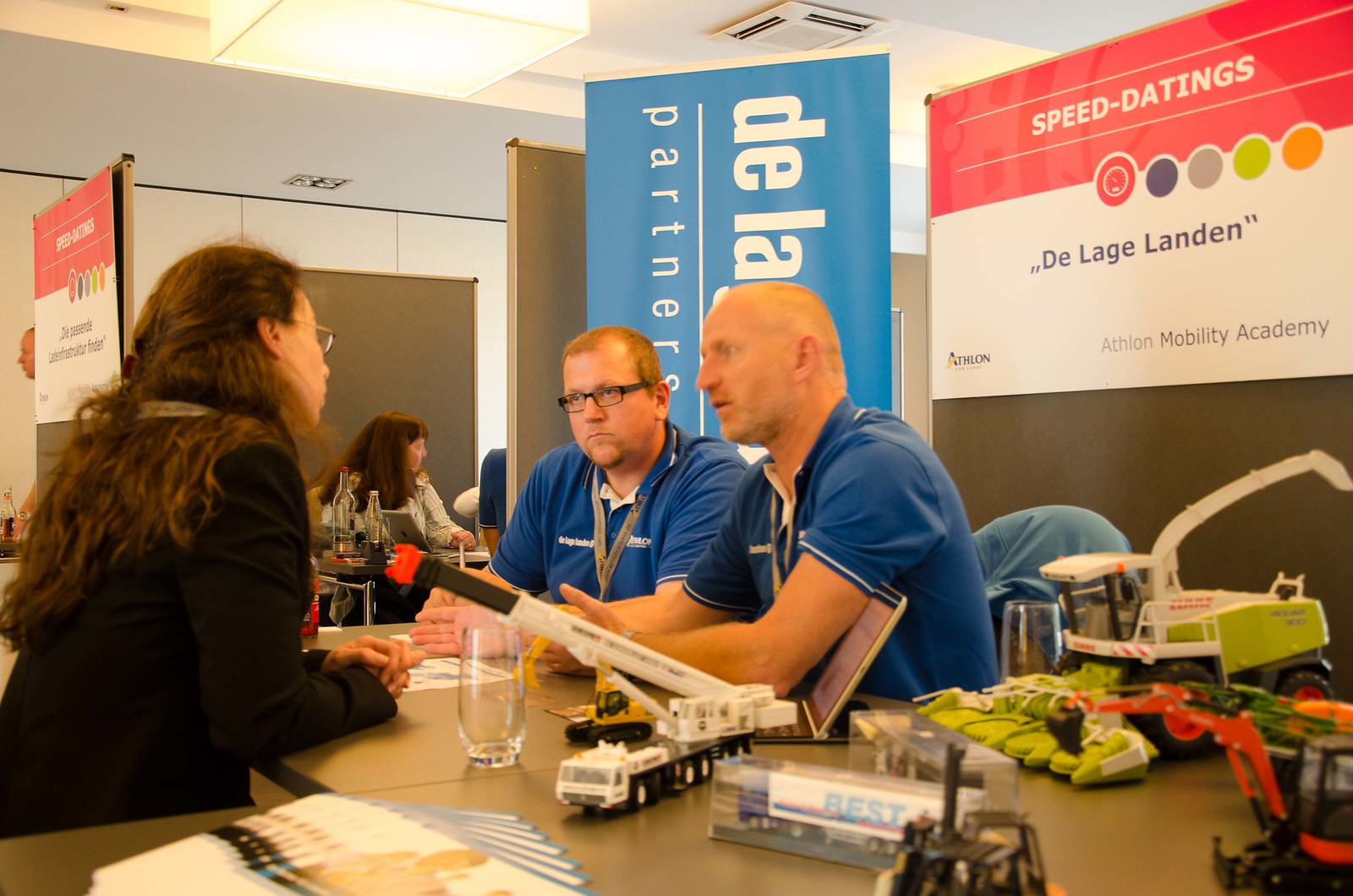The indoor image captures a meeting area or conference setup. Central to the scene are several people seated around a table, engaged in conversation. Notably, on the left side of the table sits a woman with long brown hair and glasses, facing two men in blue collared shirts at the center. One of these men also wears glasses. The table they share is strewn with various items, including brochures, a glass of water, and several miniature construction vehicles in colors such as white, green, and red.

Behind this trio, a woman with long brown hair is visible in the background. Additionally, the room features prominent signage above, with text proclaiming "Speed Dating," "DeLa Partners," and "Athlon Mobility Academy." The signs are in a mix of bold colors — blue, white, red, and sections with orange, yellow, and brown hues. Overhead, there are bright lights and air vents illuminating the space. The atmosphere and various details suggest an organized event or conference setting.